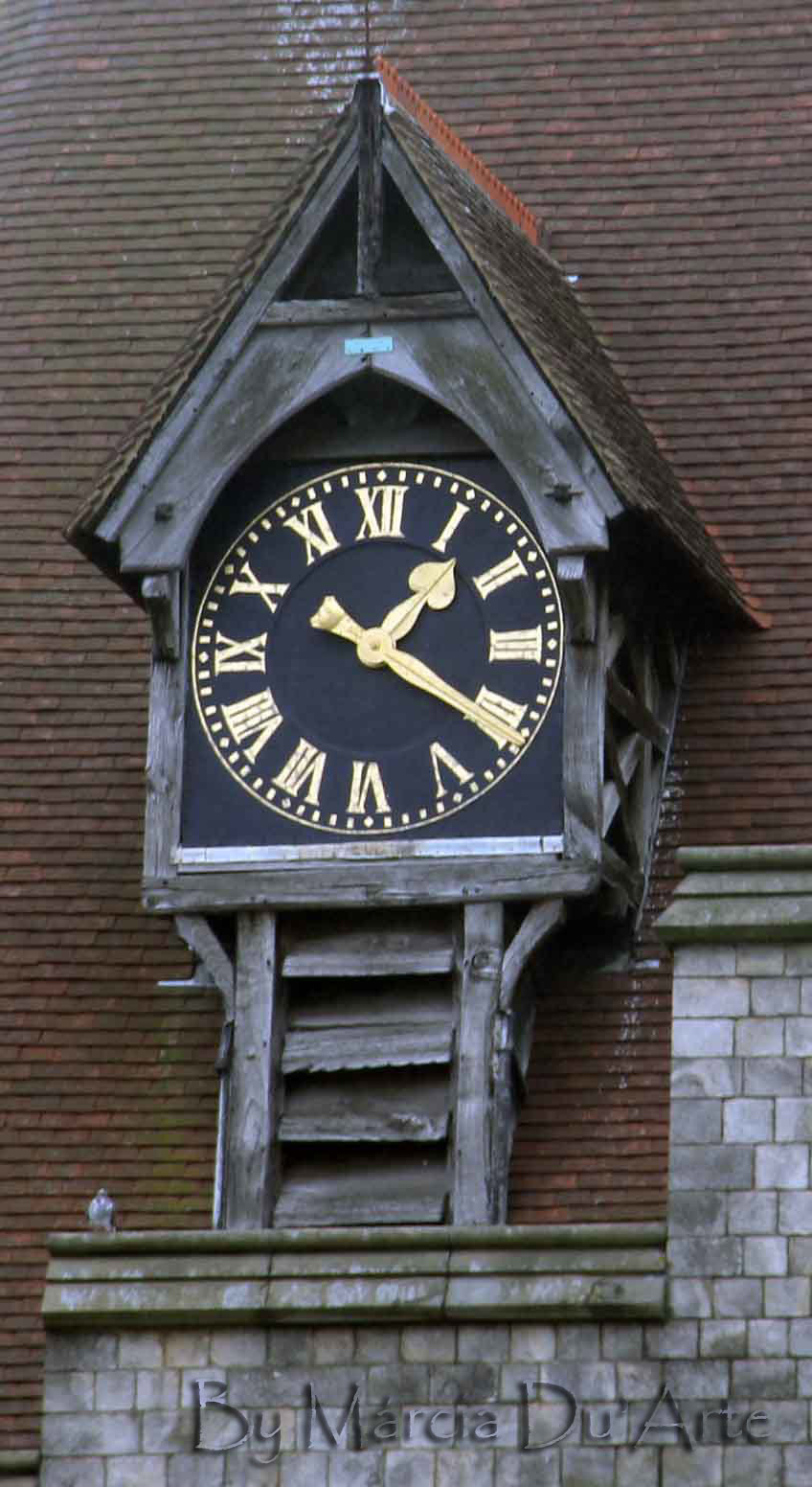In the image, a brick wall serves as the background, featuring a white brick mantel. Atop the mantel sits an elegant, vintage clock, designed to resemble a miniature house. The clock is predominantly brown with a distinct brown face, adorned with yellow Roman numerals and yellow hands, adding a touch of classical charm. The base of the clock includes four small wooden steps, enhancing its quaint aesthetic. A subtle red accent graces the top of the clock, contributing to its unique appearance. At the bottom, the name "Marcia Duong" is inscribed in gray letters, indicating the creator or owner. The overall design and details suggest the clock holds sentimental value and historical significance.